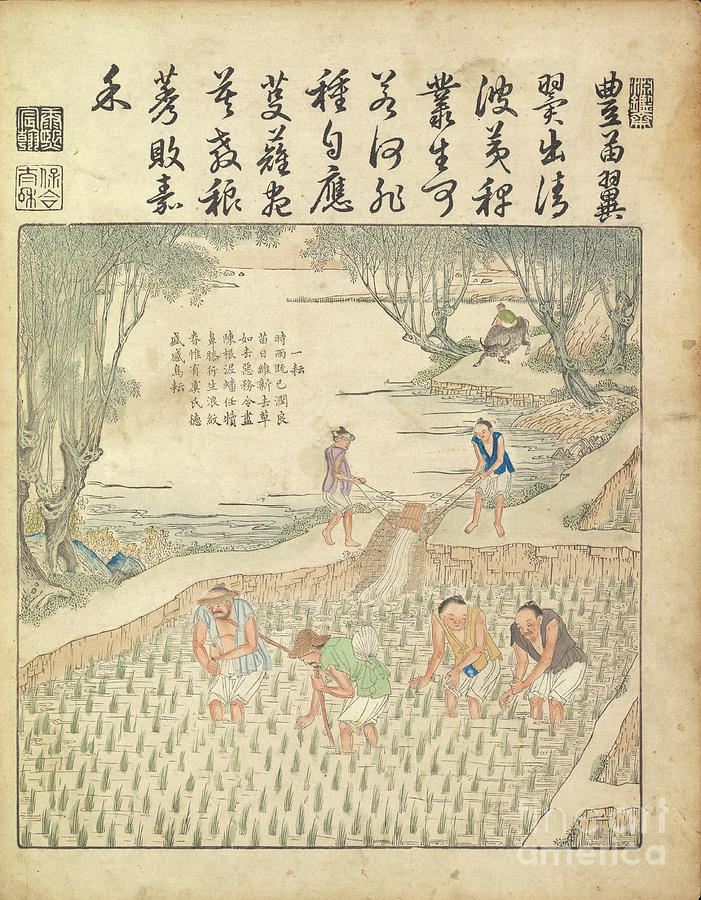This image appears to be an aged and water-stained Japanese painting or manuscript, rendered on a light brown piece of vellum. The vertically aligned, rectangular piece features three rows of hand-drawn Japanese symbols at the top, possibly text, which consists of about eight or nine characters per row. Interspersed among the text are square shapes containing additional symbols, some shaded in black and others in the lighter brown background of the vellum.

Below the text is a large, square-bordered illustration depicting an agricultural scene. The foreground shows four emaciated workers standing knee-deep in water, tending to plants in what appears to be a rice paddy. Each worker wears a mix of light blue, green, beige, and gray vests with white shorts. Two of the workers are wearing hats. In the background, two additional figures are seen emptying pails of water into the field from a bamboo gate, suggesting the irrigation of the crops. At the edges of the scene, trees are sketched, enhancing the rural setting. Also notable is a river flowing behind the figures, with a bull being ridden by someone further in the background. Fine Art America is subtly superimposed in white at the bottom right of the image.